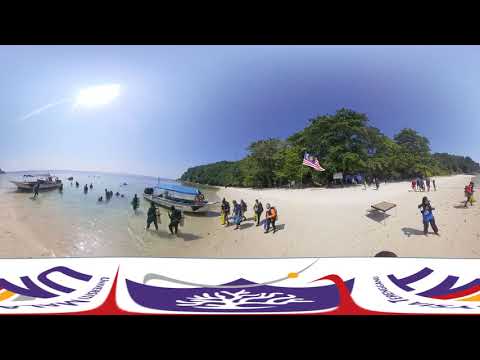This photograph captures a lively beach scene under a bright, sunny sky. The upper portion showcases a gradient blue sky with the sun shining brilliantly on the left. Below, shallow, clear waters gently meet the sandy shore, where two flat-bottomed boats with blue covers are docked. Numerous people, some gearing up with diving equipment, are either in the water or walking towards it.

In the background, a dense forest of trees lines the beach, accompanied by a flag featuring red, white, blue, and yellow hues, which appears foreign. A four-legged table is set up near the trees on the sand. 

Further details adorn the photograph: a black header and footer frame it, and above the footer, a white horizontal band with purple lettering and design elements—resembling a tent with three peaks, red waves, and the outline of a white tree—adds an artistic touch. The overall scene exudes a vibrant and international beach day.